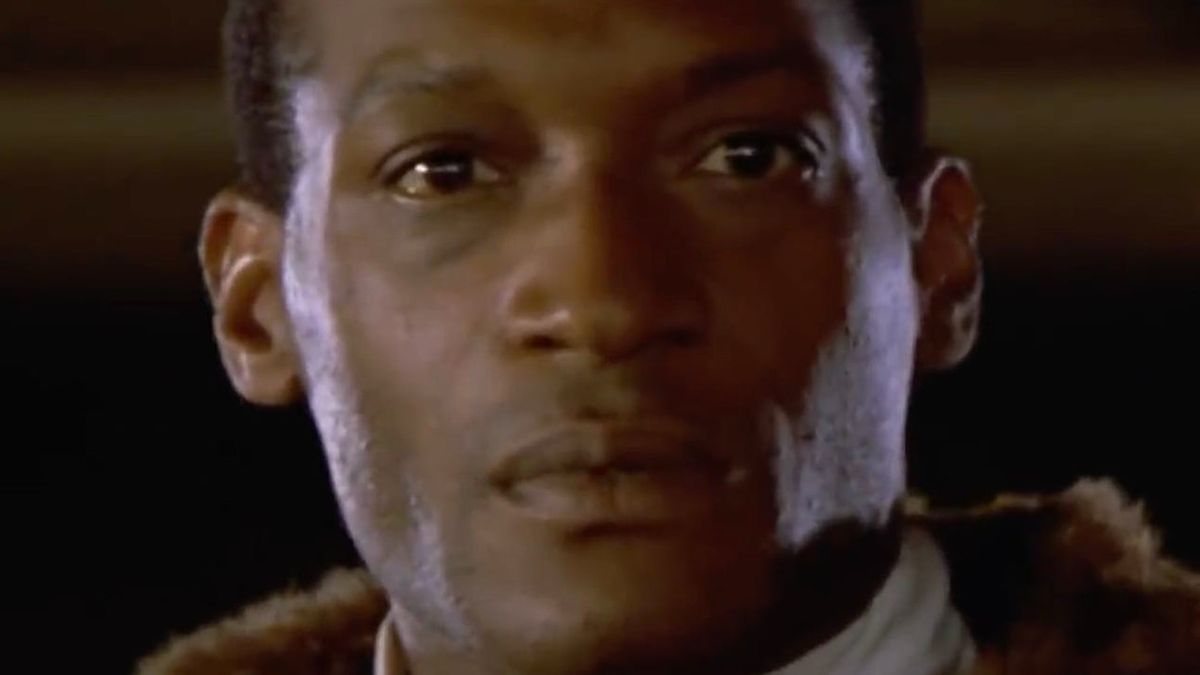The image appears to be a close-up still from a show or movie, featuring a black man with dark brown eyes and short black hair. He's clean-shaven and has distinct facial features, including a wide nose and full lips. He is dressed in a white turtleneck that wraps noticeably around the sides of his neck, particularly visible on the right, and a brown fur coat with a prominent furry collar. The lighting highlights the sides of his face, contributing to an intense look as he gazes directly at the camera, appearing upset. The background is a dark blackish-brown with a lighter brown area near the top, separated by a horizontal beige line running behind his head. The details of his face are cut off just above his eyebrows and at the very edge of his chin.